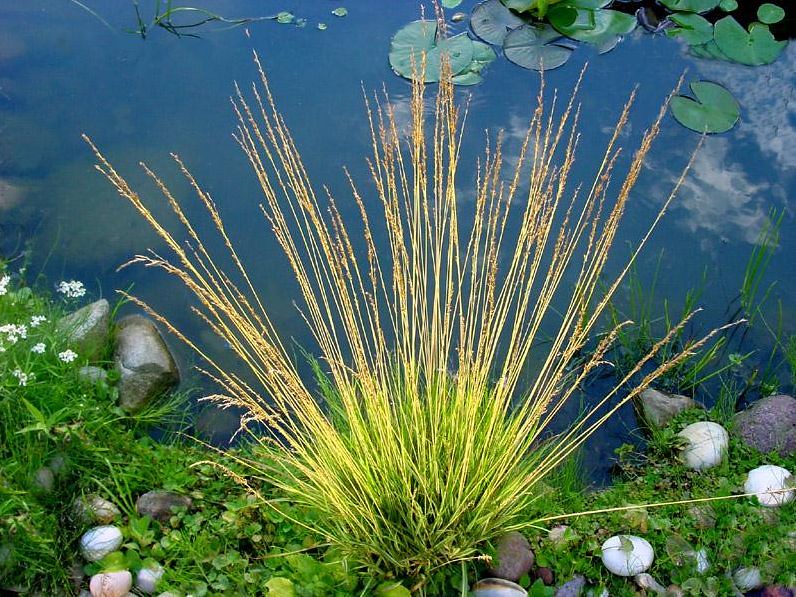This detailed photo, taken outside, focuses on the lush and vibrant scene by the edge of a small pond. Dominated by verdant greenery, the foreground features a dense mix of grass, shamrocks, and various other plants. Notably, there are large yellow weeds—or potentially aquatic weeds—that stand tall at the center of the image, resembling tumbleweeds or wheat. The scene is rich with details: numerous plants grow closely together, creating a tapestry of pointed green stems and healthy foliage. Along the pond's edge, large stones are visible both above and just beneath the surface of the water.

In the distance, the eye is drawn to a cluster of floating lily pads situated in the top right corner of the image. Clouds are softly reflected on the pond's surface, adding a serene contrast to the earthy elements. In the top left corner, partially obscured plants emerging from the water can be seen, possibly cattails, though their exact nature remains uncertain. Surrounding the pond, several stones are interspersed with moss and various other thriving plants, completing this picturesque and serene aquatic landscape.